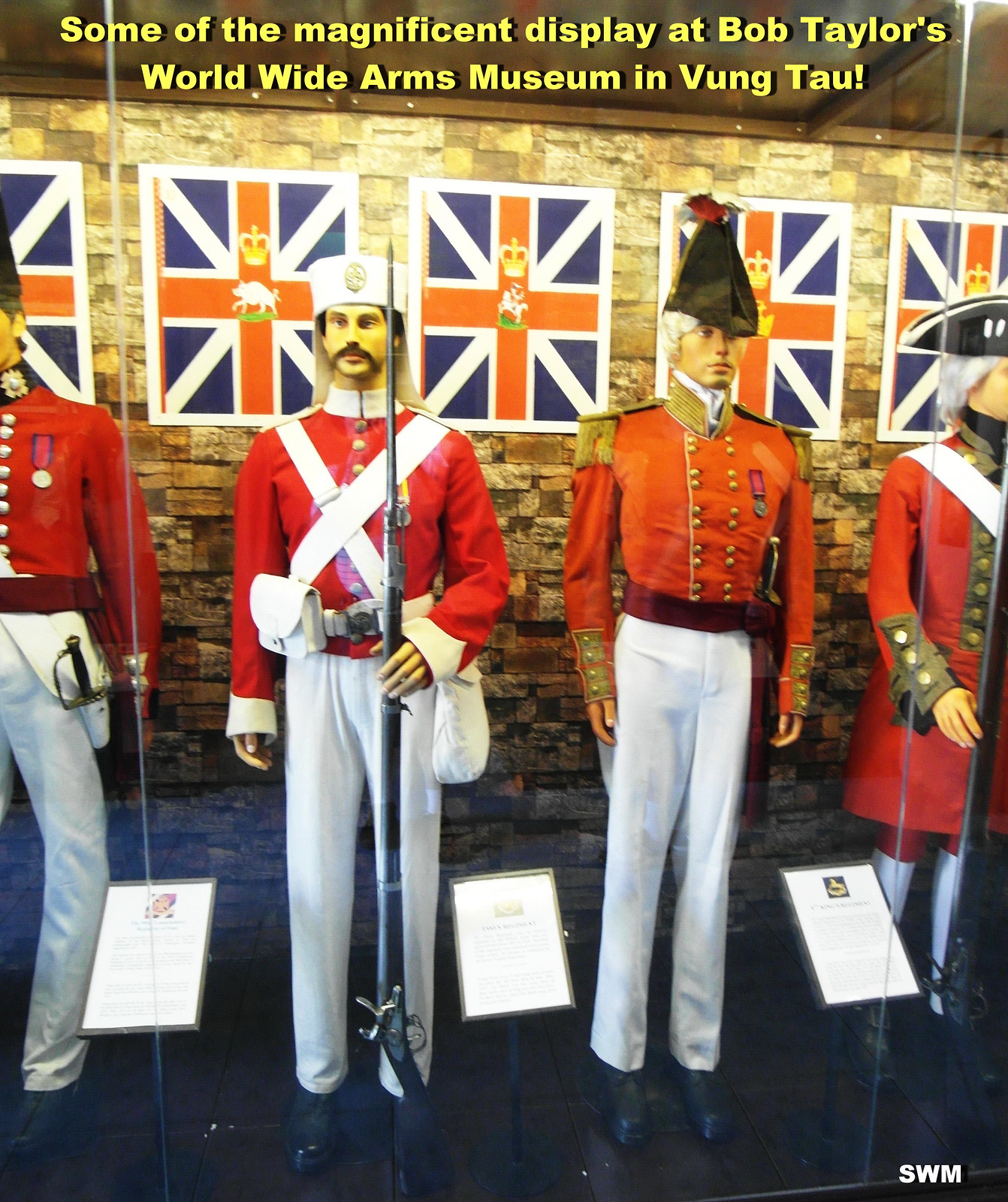The image features four life-size mannequins in a glass enclosure with a brick wall backdrop adorned with British-style flags. The prominently displayed mannequins are dressed in historical British military uniforms. The central mannequin on the left wears a red shirt and white pants, with a white hat, and brandishes a musket. His counterpart on the right, also in a red uniform and white pants, exudes authority with gold tassels on his shoulders and a distinguished black hat, although he holds nothing in his hands. Flanking these central figures are two additional mannequins, partially visible in similar red and white uniforms, but their faces are obscured. Small plaques next to each mannequin provide further information about the uniforms. Above the display, yellow text reads, "Some of the Magnificent Display at Bob Taylor's Worldwide Arms Museum in Vung Tau."